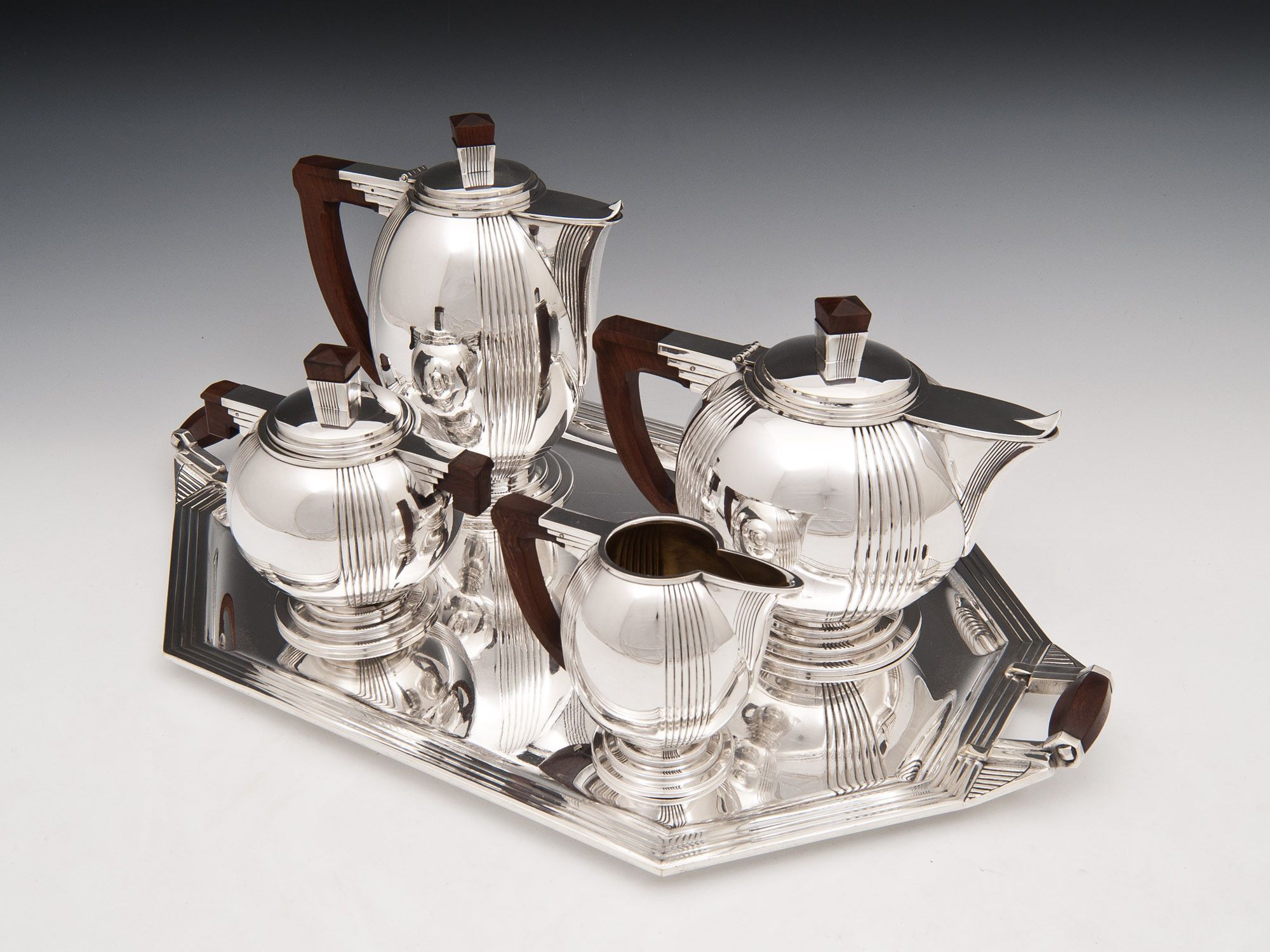In this image, we see a detailed arrangement of a silver-colored tea set displayed on a reflective silver serving tray with brown handles. The set includes four distinct pieces, each with a shiny silver finish and matching wooden handles. Three of the pieces have lids, while one does not. 

On the left side of the tray stands a tall, slender teapot designed for brewing tea, accompanied by a shorter and rounder teapot likely meant for hot water or another beverage. To the right of these, we find a smaller pot, typically used for sugar, and the smallest piece, a creamer, which is the only one without a lid. Each item reflects beautifully on the tray, creating a cohesive and elegant display. The background of the image is contrastingly white and black, highlighting the meticulous design and polished finish of the tea set.